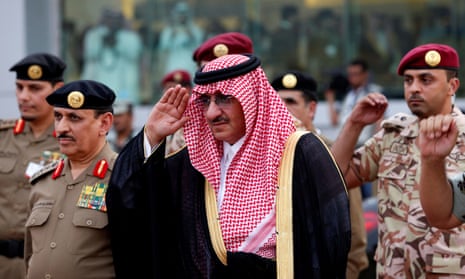The image captures an outdoor scene in a Middle Eastern country featuring military personnel and a significant figure. At the center stands the former Saudi Crown Prince, now deposed, dressed in a black robe with gold accents and a red and white checked headscarf held in place by a black agal. His hands are raised, and he wears glasses, suggesting his importance. Flanking him are several military members: to his right, soldiers in camouflage uniforms with maroon berets, adorned with gold patches, and to his left, soldiers in brown uniforms showcasing their ribbons, with black berets also featuring gold patches. All the military members are saluting with their right hands. The overall composition is realistic, with a focus on the central figure and his surrounding entourage, set against a blurred backdrop.